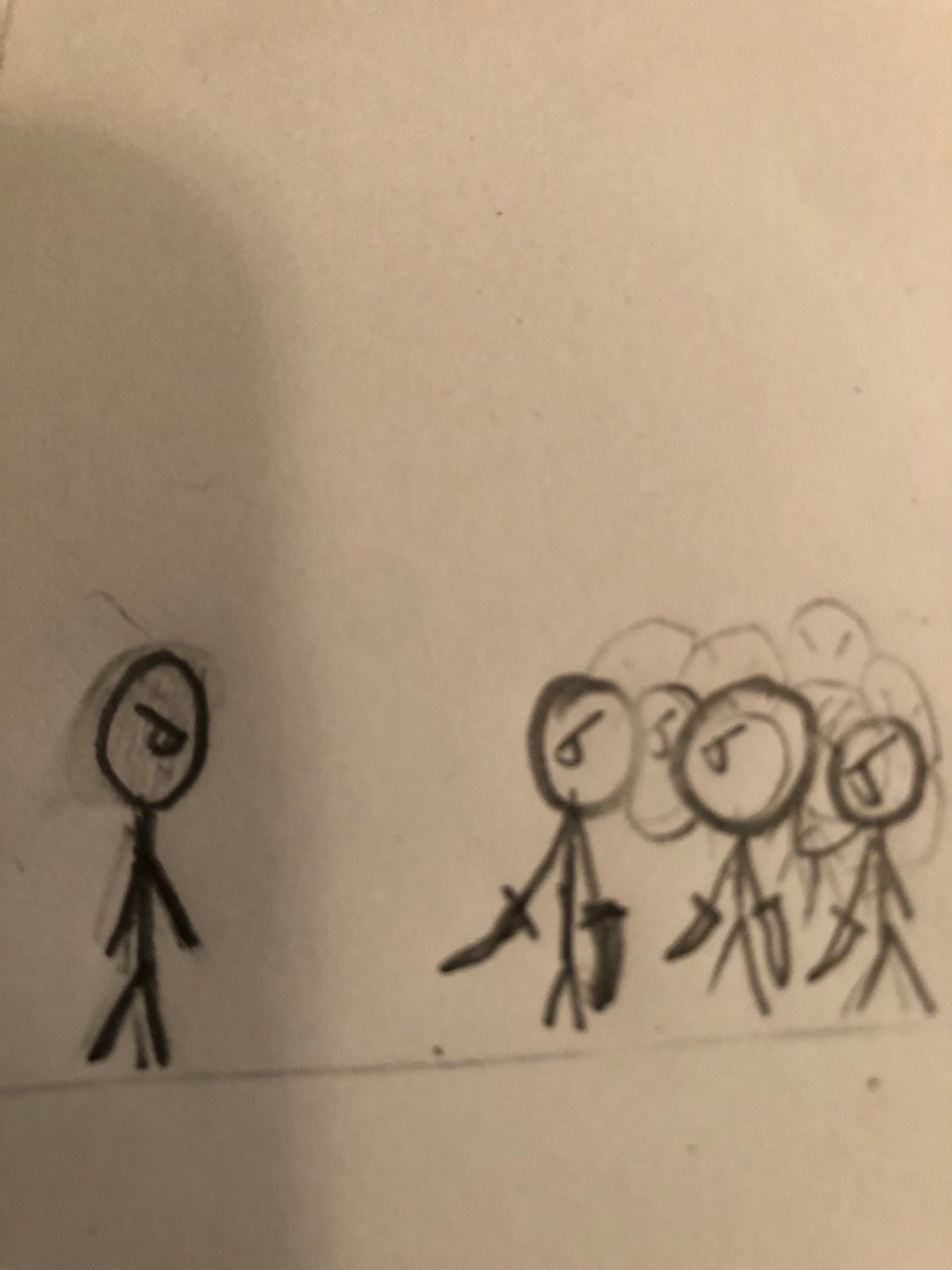On a white background, a lone stick figure stands on the left side of the image, exhibiting an angry expression and casting a shadow. This figure looks down to the right, seemingly perturbed. To the right, a mob of stick figures advances, each brandishing swords. The stick figure at the forefront of the mob wields two swords, one in each hand, while the figure behind them also holds two swords in a similar manner. All the figures in the mob wear simplistic, angry faces, reflecting their collective rage. The background is predominantly white with minimalistic details, such as darker shadows on the left and some spots on the ground. The figures in the mob are darkly shaded in contrast to the lighter shading of the figures in the background, enhancing the dramatic tension of the scene.